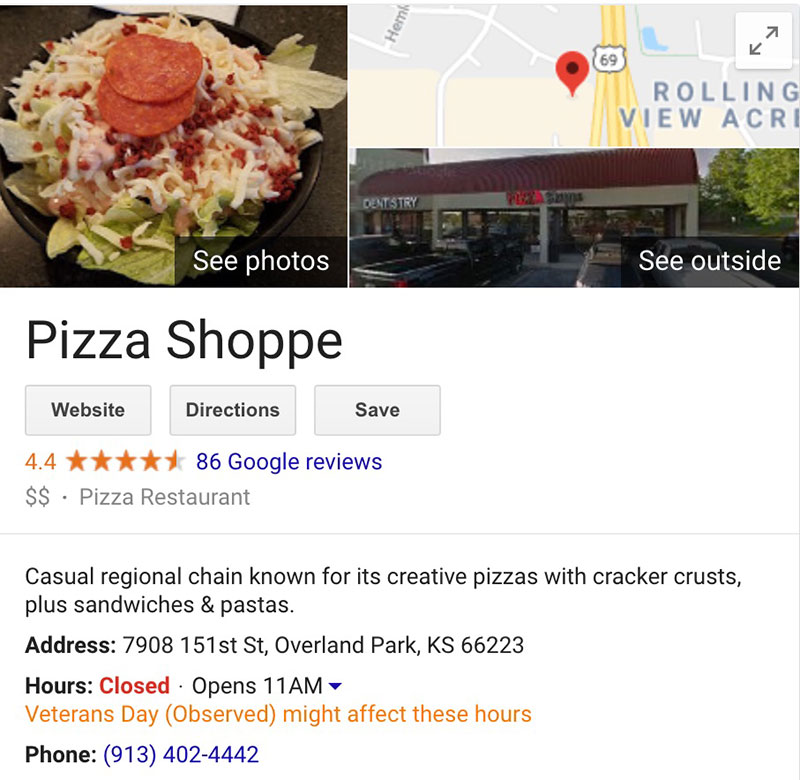This detailed caption describes a business's Google page:

The top left corner displays an appetizing image of a salad, adorned with fresh lettuce, shredded cheese, pepperoni slices, and crispy bacon bits. At the bottom right of the page, there is a prompt labeled "See photos." Adjacent to this, on the right, sits a map with a red pin marking the business's location. Below the map is an exterior photo of the storefront, accompanied by a "See outside" option at the bottom right.

Beneath this, the business is identified as a "Pizza Shop," featuring three grey buttons labeled "Website," "Directions," and "Save." The shop boasts a rating of 4.4 stars out of 5, highlighted in orange, with 86 Google reviews. The listing further indicates the business's price range with two money signs and categorizes it as a "Pizza Restaurant."

A descriptive blurb follows, noting that this is a casual regional chain celebrated for its inventive pizzas with cracker crusts, as well as its offerings of sandwiches and pasta.